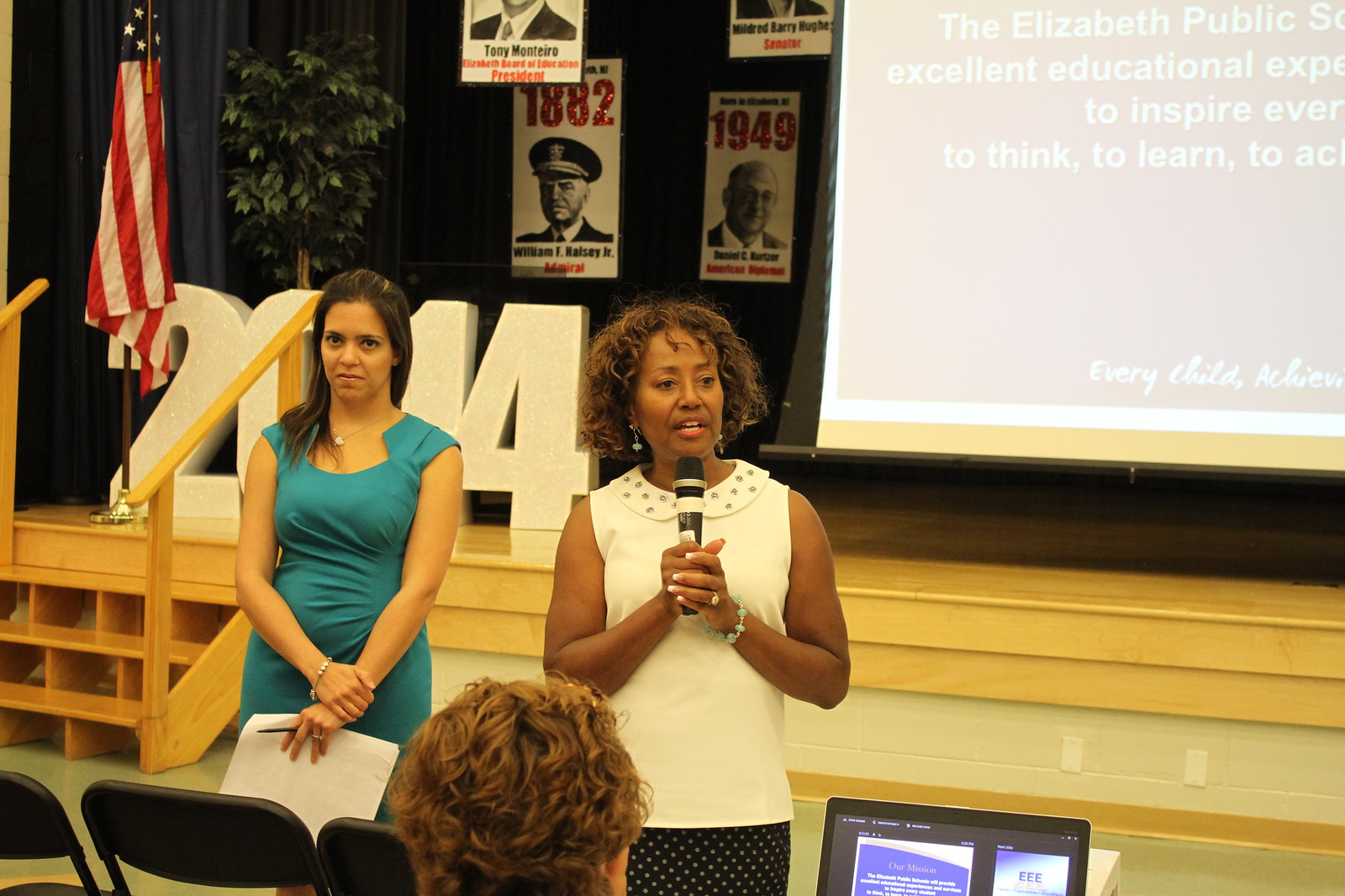This photograph, taken in landscape orientation, captures an event, likely a conference, centered around two women on a wooden stage. The focal point is an African American woman standing in the middle, holding a microphone with both hands as she speaks. She is dressed in a short-sleeved, white-collared shirt paired with a black and white polka dot skirt. To her left stands another woman, possibly Hispanic, holding a piece of paper and a pen. She is dressed in a blue or bluish-green dress and maintains a straight-faced expression while looking at the camera.

The stage backdrop features large lettering spelling out "2014," accompanied by an American flag. Posters with various dates and portraits of notable men, presumably leaders, adorn the background. In the upper right-hand corner, a projection screen displays white text. In the foreground, at the bottom of the screen, a few chairs are visible alongside the back of an audience member's head, who appears to be managing the laptop that controls the projection screen cues.Overall, the image conveys a formal atmosphere with an organized setup, emphasizing the speaker's role in addressing the audience.